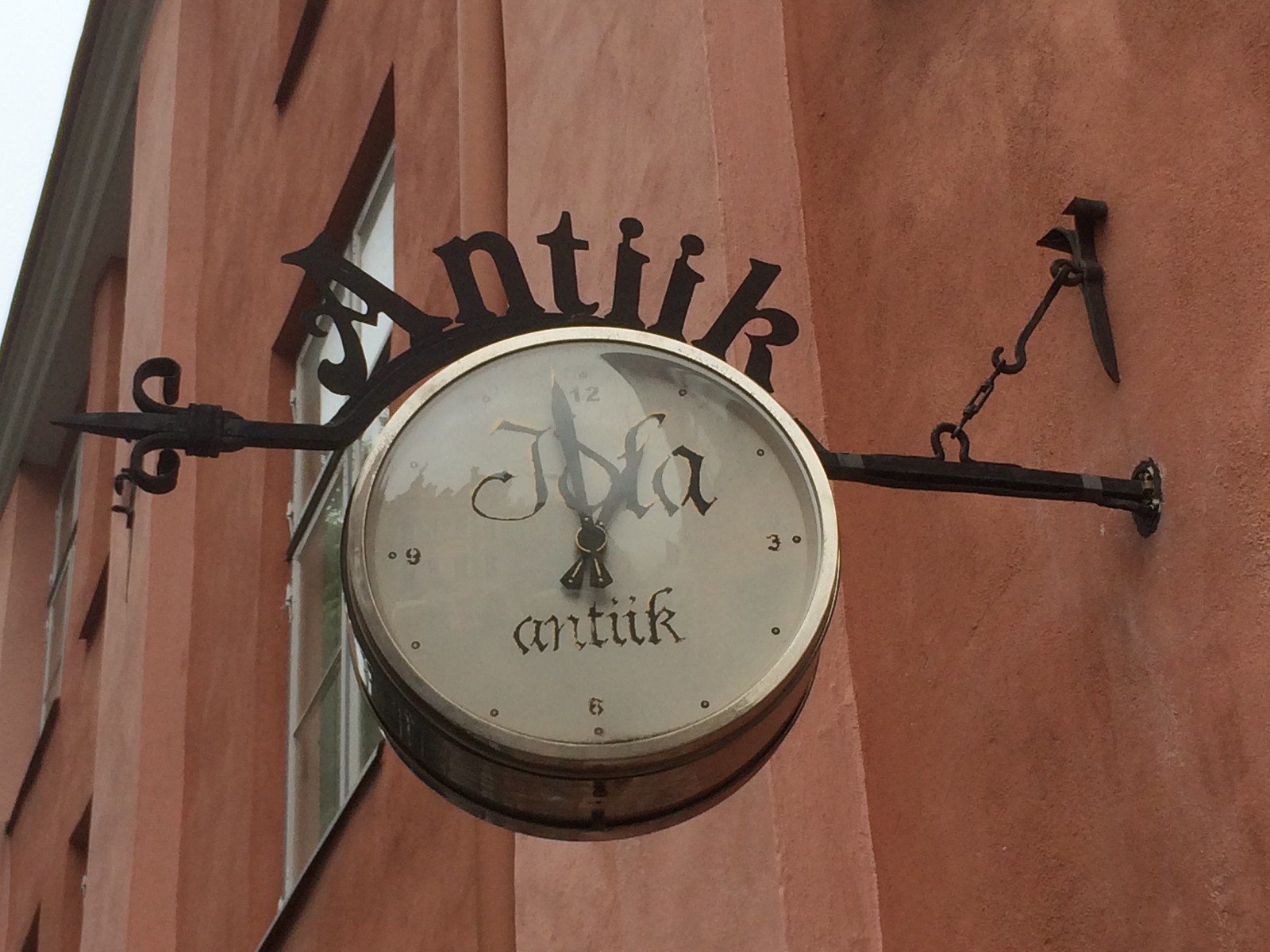This photograph captures the exterior of a rust-colored building, likely in northern Europe, featuring alternating panels of red and rosy pink. Attached to the wooden wall is an antiquated outdoor clock, mounted on a black metal beam and iron hooks. The beam, which protrudes horizontally, is adorned with metal letters spelling out "ANTIIK," suggesting a possible antique shop. The clock has a white face with black, old-fashioned stencil numerals 12, 3, 6, and 9, and it displays the time as almost 1 o'clock. The face also features the words "Jofa Antique." The clock’s design, reminiscent of a weathervane, includes a fleur-de-lis-like spike and a single chain link for additional support. The surrounding area includes visible windows, resembling apartment windows, providing a quaint, charming backdrop to this vintage timepiece.